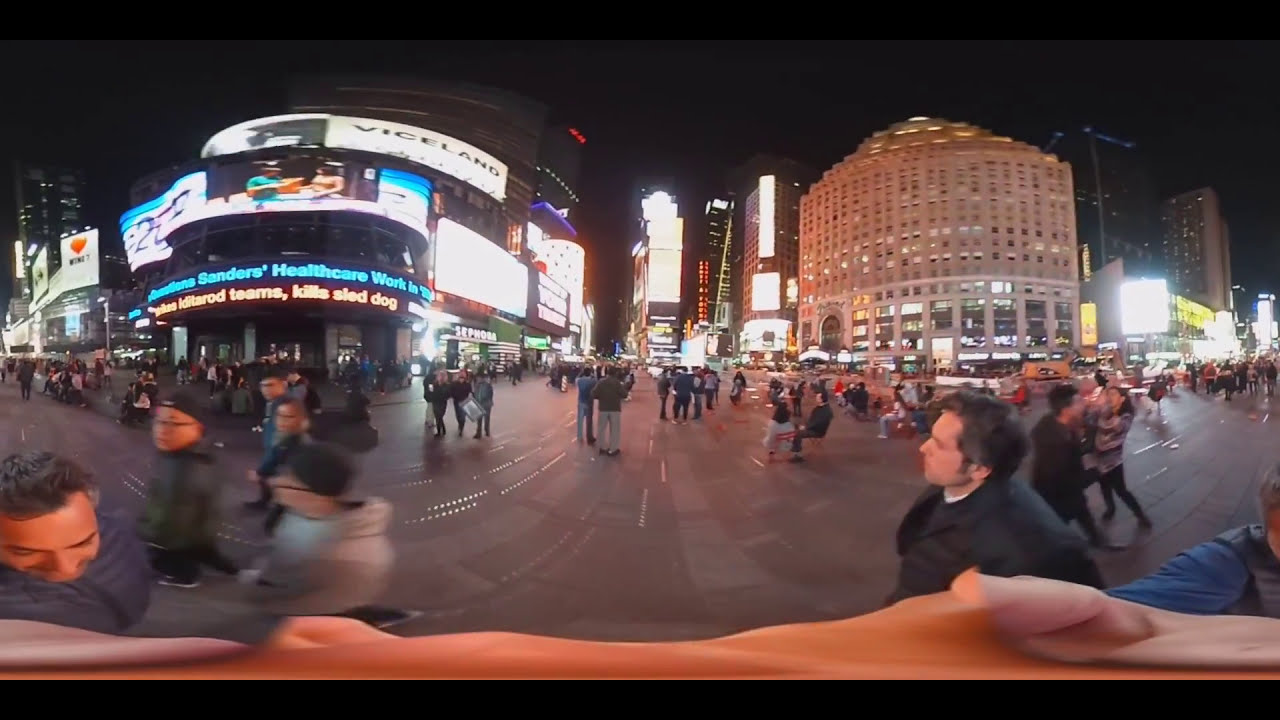This nighttime urban scene, possibly in a busy city center like New York's Times Square, is captured with a fisheye lens that distorts the buildings, road, and people, giving the image a slightly surreal look. Skyscrapers illuminated with various advertisements and billboards dominate the background, with a prominent scrolling news feed in English mentioning "Sanders Healthcare" and an intriguing message about a "rod team kills sled dog." A red heart is also visible in the illuminated text. The scene shows a mix of black, blue, white, and tan buildings, including a distinctive cylindrical one with many windows. 

The image seems to be taken from the middle of a road, which is closed to traffic as no cars are visible. People are scattered around, many taking photos, suggesting that an event might be taking place. Notably, the camera itself is visible, with a distortingly wide shot capturing the hand of the person holding it at the bottom of the image. The crowd includes individuals in a variety of coats and pants, details such as a blue coat, green coat, black cats, glasses, and hoodies adding to the vibrant human activity. The sky is pitch black, contributing to the ambiance created by the artificial lights and advertisements, with no stars, clouds, or moon visible.